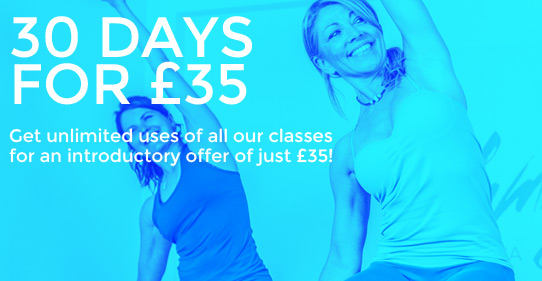The advertisement features a vibrant turquoise blue background, providing a calming and inviting atmosphere. Overlaying this background are several images, some shaded in darker turquoise tones, adding depth and contrast. In bold white letters at the center of the ad, it prominently displays the offer: "30 days for £35." Below this, also in white text, is an enticing invitation: "Get unlimited access to all our classes for an introductory offer of just £35!"

To visually enhance the offer, the ad includes images of two women, each engaging in a stretching pose. On the left, a woman with dark hair and wearing a dark-colored tank top stretches to her left. To the right, another woman with blonde hair in a ponytail, donning a white tank top and a necklace, mirrors the first woman's stretch to her right. The turquoise hue overlays these images, integrating them seamlessly with the background and maintaining a cohesive color theme.

Behind the stretching women, a partially obscured logo hints at the branding of the fitness establishment, though the text is mostly hidden behind the figures, adding an element of intrigue. The overall design emphasizes the promotional offer while subtly showcasing the brand's identity and the active, health-focused lifestyle it promotes.